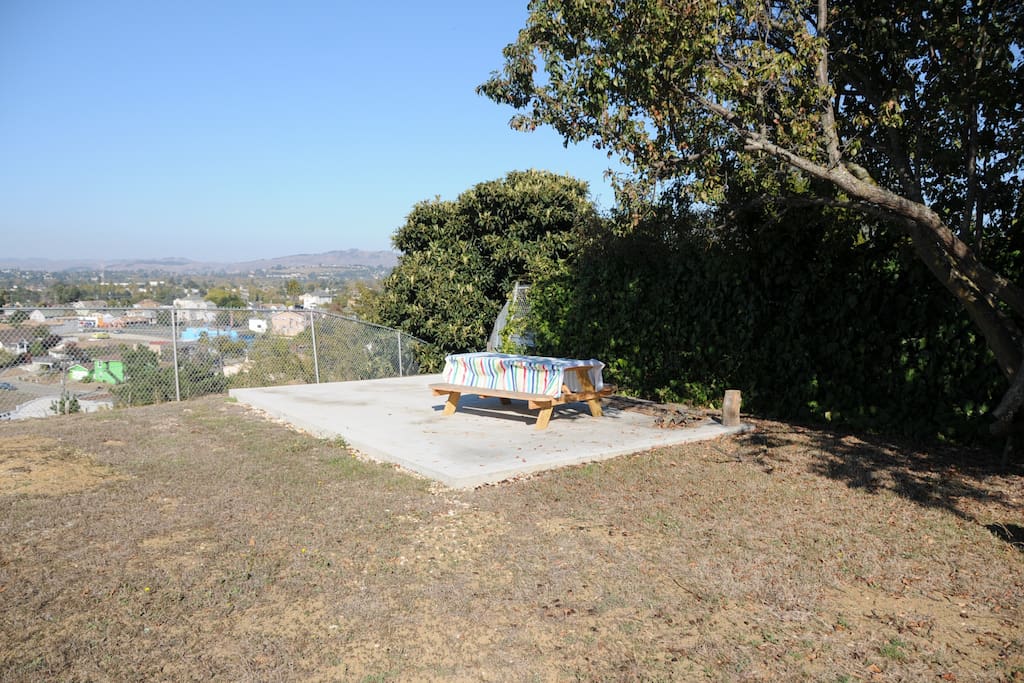In this image, we are presented with an outdoor scene dominated by a central wooden picnic table situated diagonally on a large, light gray concrete block. The table is adorned with a vibrant, multicolored striped tablecloth. The area around the table appears dry, with sparse and brownish grass. On the right side, there are dense clusters of trees adding to the natural feel of the scene. To the left, a short metal fence hints at the elevated position of the picnic area, providing a view of the flatter grassland extending towards the horizon. In the distance on the left, you can spot several houses and other buildings, which gradually give way to rolling hills under a clear blue sky. The combination of these elements suggests a serene yet somewhat dry and barren environment designed for relaxation and outdoor dining.